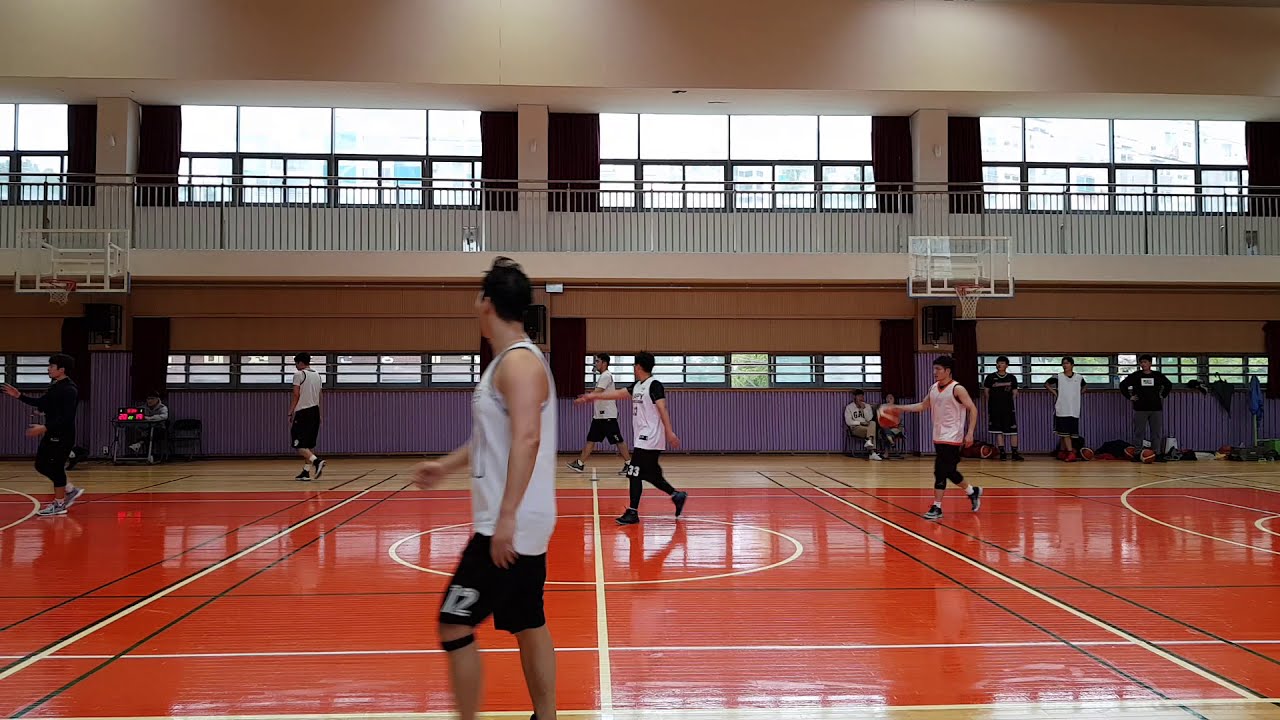The image depicts an indoor basketball gym where a group of players, wearing white jerseys with black shorts, are engaged in a game or possibly a practice session. The scene is centered on an orange and light wood-colored basketball court that occupies the bottom half of the image. White and black lines demarcate various sections of the court. Five players are scattered across the court, with one visibly dribbling the basketball. The players, who appear to be of Oriental descent, are positioned in a manner that suggests the game is currently in play. A coach, dressed in a black long-sleeve shirt and black pants, is likely supervising the activity from the side.

Above the court, a horizontal purple wall splits the image. Above this wall, the backboard of the basketball hoops is white with orange rims. At the top of the image, a gray balcony with windows, each having about four panes, overlooks the court. Additional black detailing is visible around the windows. The setting is quite vibrant, featuring colors like red, white, black, tan, gray, blue, and the distinct purple of the wall. People are also seen on the sidelines, with some standing and others seated in chairs. The polished and somewhat shiny floor suggests a well-maintained gym, emphasizing an atmosphere of active engagement in the sport.